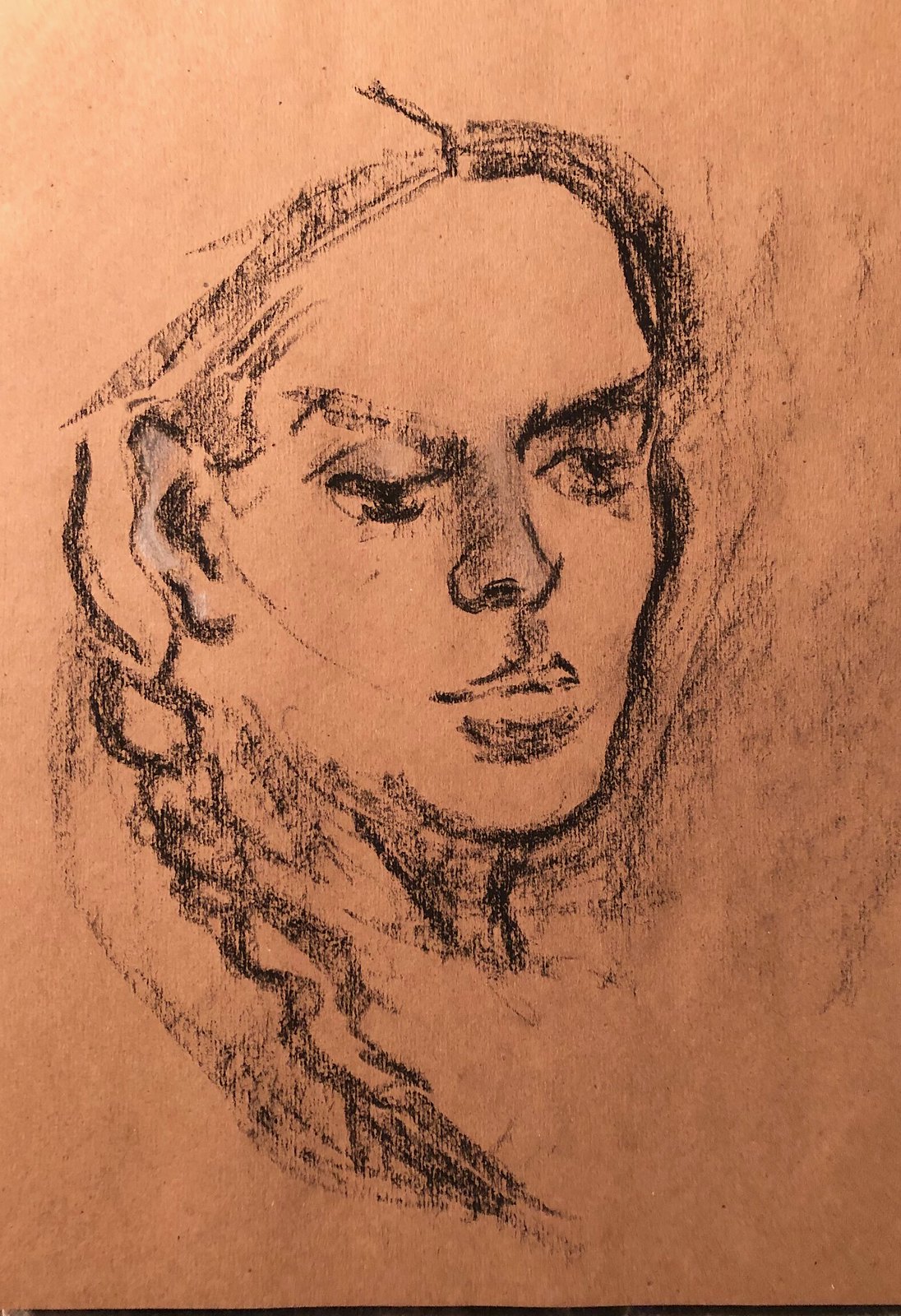The image is a photograph of a charcoal drawing on a rough, dark brown-orange piece of paper. The drawing is centered and detailed, featuring the face of a woman. Her hair is parted in the middle with wisps falling on the left side and a braid cascading over her right shoulder. Her right eyebrow is raised, and she has half-lidded eyes with blue shading on her right eyelid. The nose is prominently shaded and there's a defined philtrum above her indented top lip. Her lips are plump and she has a strong chin and cheekbones. The side of her head is slightly visible, revealing a pointed ear highlighted with white. The sketch is heavily shaded, giving it a realistic and textured appearance, likely done with black charcoal or pencil, suitable for an art class assignment.